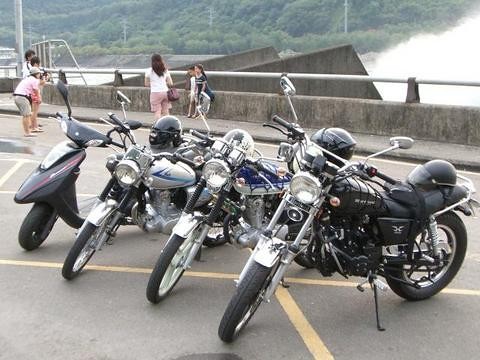In this vibrant image, a picturesque scene unfolds beside a highway at a pull-off area where three large motorcycles and a smaller electric scooter are parked diagonally. The motorcycles, possibly BMX style, are joined by a scooter reminiscent of those often used by women. The parking area, though loosely defined with yellow lines, serves as a convenient spot for this group. Resting on the bikes are helmets, hinting at a recent ride.

The backdrop features a dynamic dam with foam-laden water crashing against a stone structure that slopes upward and then sharply down. Metal rails affixed to a concrete base ensure safety for onlookers, who are scattered across the area, savoring the view. Amidst this scenery, multiple people, possibly families, are visible. One woman, distinguishable by her white T-shirt and pink shorts, is taking a photo of two little girls. Nearby, another woman with a pocketbook is accompanied by two men in casual wear—one in a pink shirt and grey shorts—adding to the relaxed, joyous atmosphere.

Behind them, the rough waters of the dam contrast with the tranquility of the surrounding trees and clear sky, creating a stark yet beautiful natural setting. This lively moment captures a day of exploration and leisure, highlighting the interactions of the people present as they revel in the beauty and excitement of the environment.